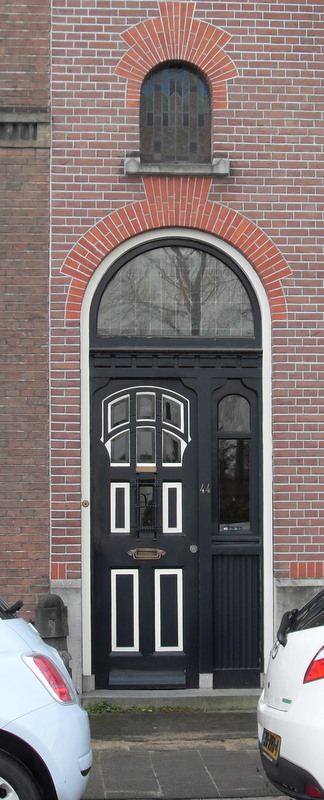This is an outdoor, daytime street view of a red brick building, focusing on a black door set within an imposing archway. The door is rectangular and vertically oriented, with detailed features. You are standing behind a small parking area with a white car, seen from the front on the left and the back on the right. The concrete of the parking spot is visible between the cars, leading to the door.

The black door, framed by a gray concrete block at its base, dominates the scene. It features three small windows at the top and three underneath, all outlined in black with a yellowish surround. Further down, two vertical rectangles outlined in white flank a central metal slot. Below this slot, a white rectangle with black interior extends almost to the door’s base. To the right of the door is an oblong window, with its lower half dark blue.

Above the door is a large, semi-circular window resembling a sun, partially obscured by the structure above. The red brick façade of the building, characterized by its archway and sturdy construction, provides a vivid backdrop to the intricate door and its surrounding elements.